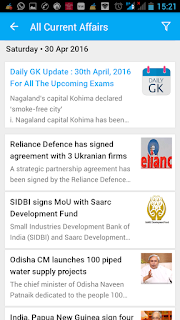Set against a solid white background, this somewhat blurry screenshot appears to have been taken from a cell phone. At the top of the image is a banner featuring a menu of icons, which are slightly difficult to discern. Notable icons include a telephone icon on the upper right, a red square icon, and a yellow icon with a blue triangle on top. The battery icon indicates that the cell phone has a nearly full charge. In the upper right corner, the time seems to be 15:21, though it is blurry.

Beneath this, there is a blue banner with white text reading "All Current Affairs," accompanied by a left-pointing arrow. The date "Saturday, 30th of April 2016" is displayed below against a gray background. Following this, within a white box, text reads: "Daily GK Update, 30th April 2016 for all the upcoming exams."

The next segment, also in a white box against the gray background, states: "Reliance Defense has signed agreement with three Ukrainian firms." To the right, there is a gray icon or box with partially visible text suggesting the word "Elliance," possibly part of the word "Reliance." Below this, in black text, it reads: "SIDBI signs MOU with Sark Development Fund."